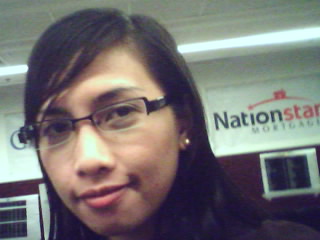The photograph captures a close-up view of a woman with long hair, wearing black-rimmed glasses and silver studded earrings. She is looking directly at the camera and smiling. The background reveals a detailed indoor setting with a white drop-down ceiling featuring a long fluorescent strip light. The far wall is painted red and features a black rectangle sign decorated with multiple lines of illegible white text. Accompanying the décor are black squares on the left side of the wall, each containing white tables. Prominently displayed on the back wall is a banner with the words "nation" in black, "star" in red, and "mortgage" in black, detailing the context of the setting.